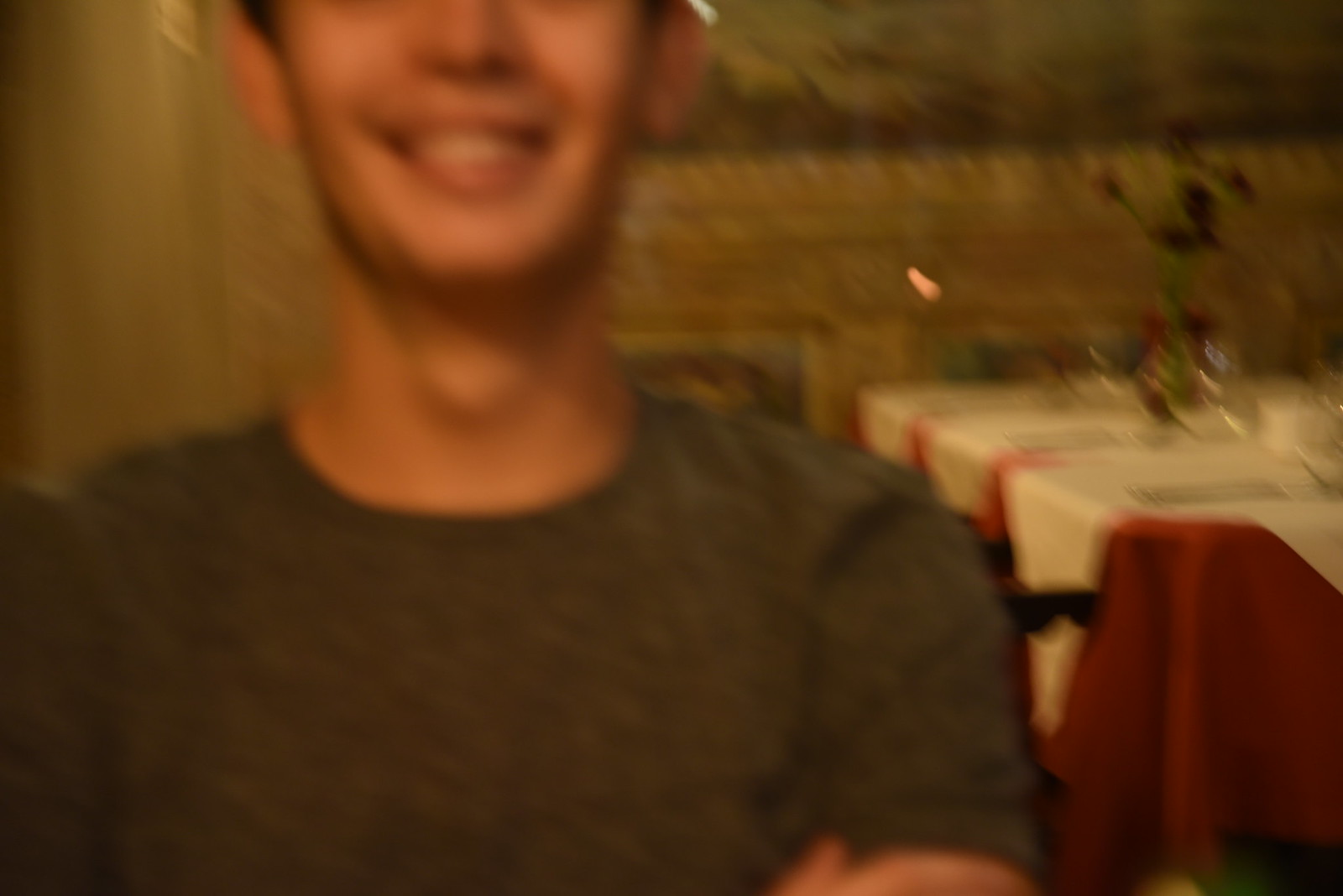The image portrays a slightly blurry scene of a man seated in a restaurant. The man's face is partially visible from the nose down, with the top of his head cut off by the image frame. He appears to be Caucasian with brown hair and slightly protruding ears. A warm smile graces his face, and he has a slender build. He is dressed in a short-sleeved gray shirt with a U-shaped neck.

The ambiance of the restaurant features beige walls, and behind the man, there is an oil painting of a landscape. A table, covered with a white tablecloth and adorned with an orangish-red cloth, is also visible. This table sports a glass vase containing what seem to be red roses with green stems artistically twisted inside. Additionally, there are partially visible, ornate gold-framed artworks adding to the room's elegant décor.